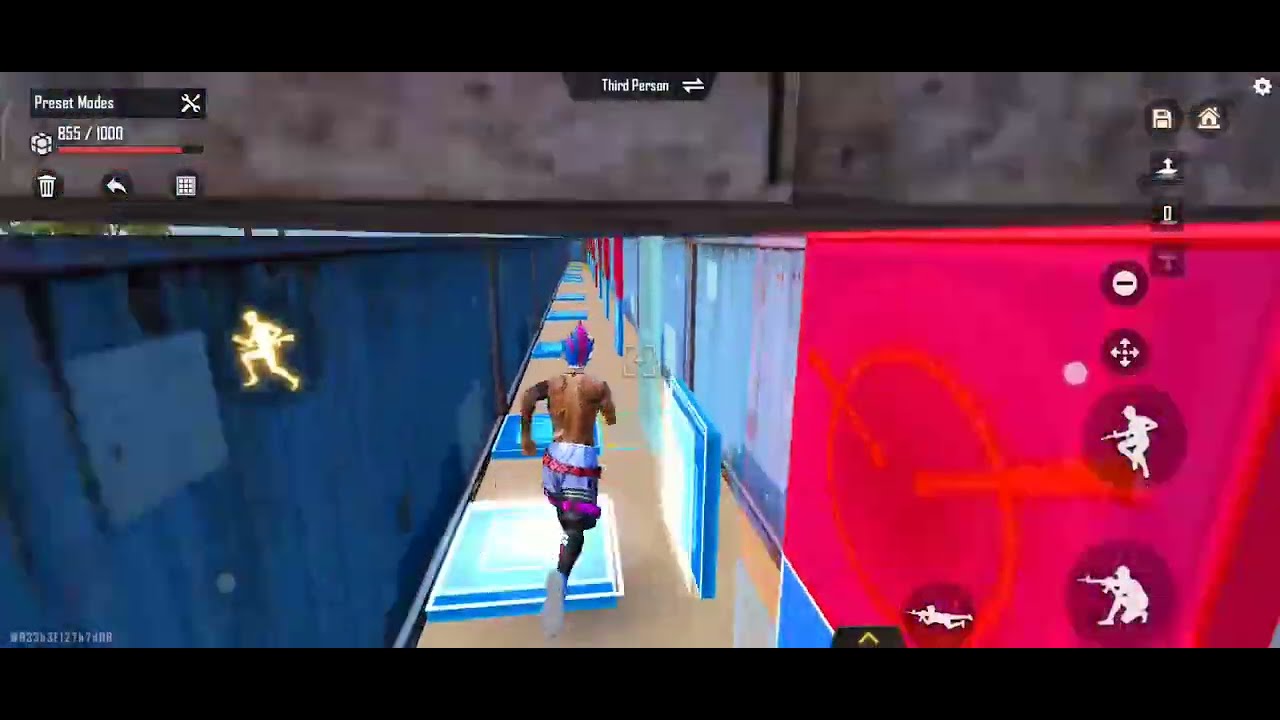In this highly detailed screenshot from a third-person shooter video game, we observe a black male character with striking blue and purplish spiked hair, mid-run down a pixelated hallway reminiscent of a shipping container area. The character is shirtless, with several tattoos visible on his left arm, and is wearing vividly colorful shorts, described variably as blue with pink flowers, or purple and blue board shorts. The hallway features a tan floor with large square blue lights, and blue and red panels lining the walls, creating a visually dynamic environment. Overlaid on the screen are various icons and HUD elements: a health meter labeled "preset modes" in the upper left corner, and along the right side, it displays a save icon, home button, and silhouettes of different action poses such as a sniper lying down or crouching. Additionally, there appears to be a secondary character off to the left, described as golden and possibly falling down a hole. This rich amalgamation of elements depicts a fast-paced moment within the game, characterized by its vivid graphical detail and dynamic in-game interface.